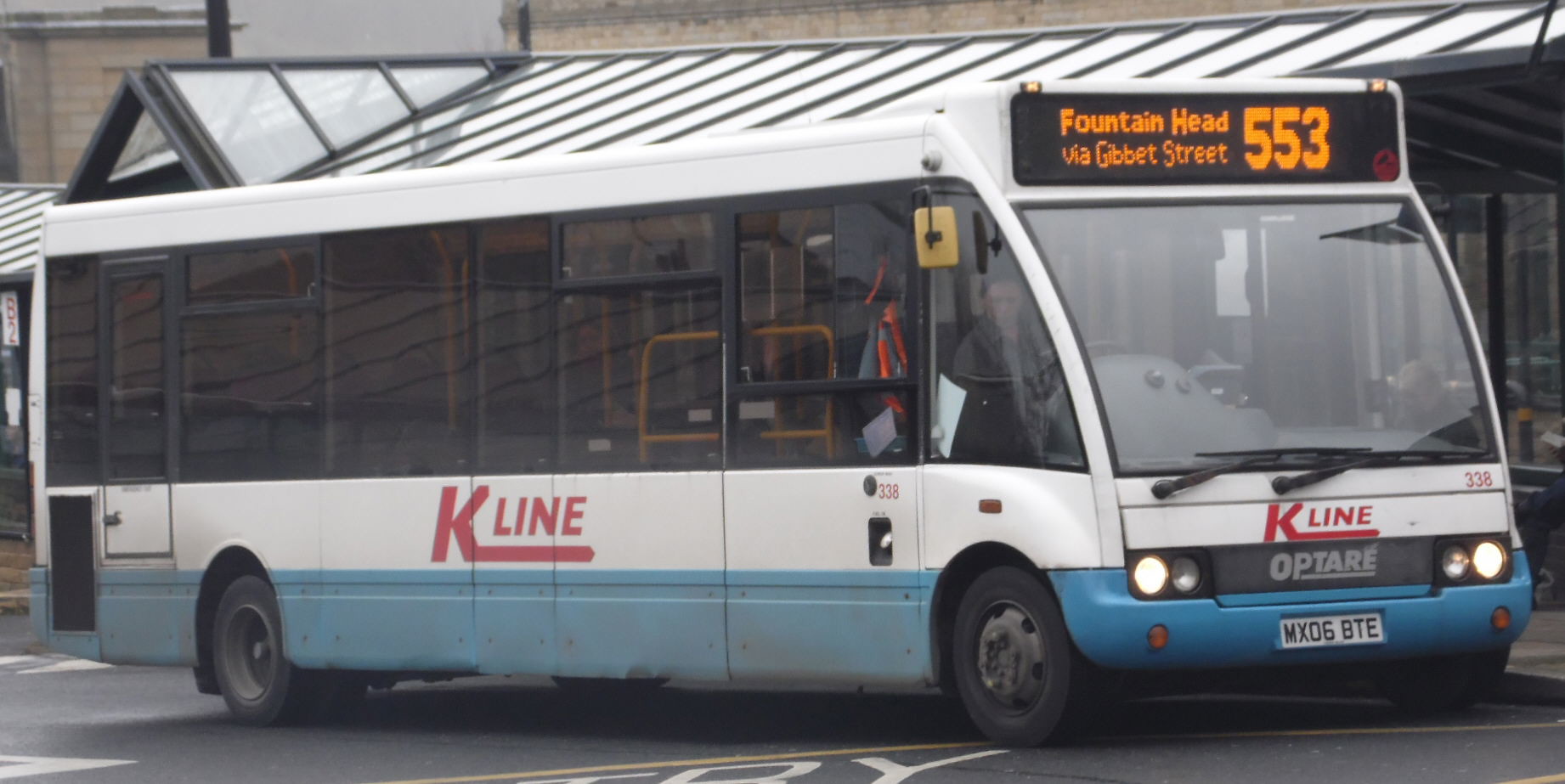The image depicts a long, stretchy charter bus predominantly white with a blue bar along the bottom. The bus, facing right, features the word "Kline" in red lettering on its side and front, with "Optare" underneath the front logo. It also bears a European license plate reading M-X-O-5-B-T-E. The bus marquee displays "Fountainhead via Gibbert Street 553" in vivid orange lettering. The photo captures the bus seemingly in a parking spot, possibly at a bus terminal or station, given the presence of a metal awning and a beige-ish tan brick or stone structure on the right. Behind the bus, part of a building with a glass roof is visible. In the foreground, letters embedded in the pavement conclude with "R-Y." The overall atmosphere is somewhat gray and overcast.